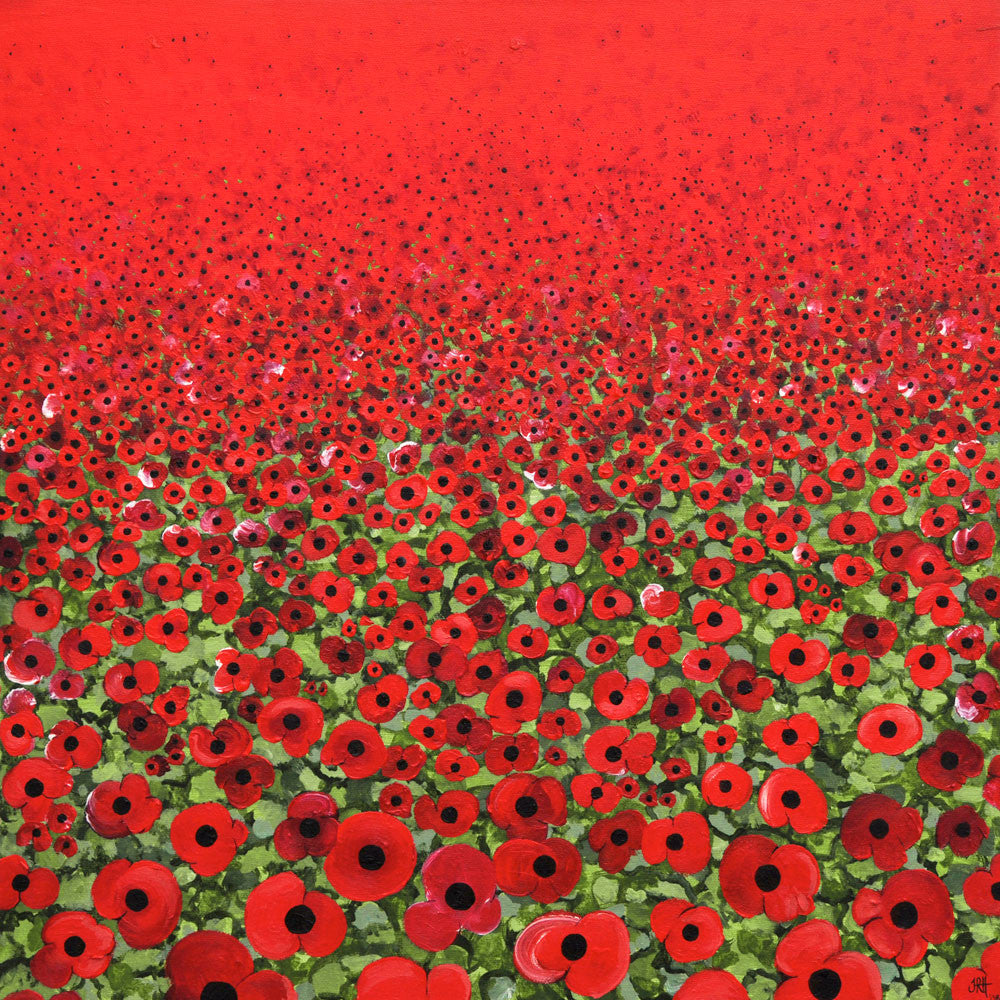This painting presents a square, vibrant field of red flowers under bright natural light. Dominating the scene are flowers with striking red petals, each featuring a distinctive black center and complemented by green leaves. The composition masterfully shifts from a close-up view at the bottom, where individual flowers and their intricate details are clearly visible, to a blurred expanse of dense red at the top, suggesting a distant perspective. This transition creates a gradient effect where the flowers appear to merge into a sea of red and black as they recede into the background. The primary colors in this detailed and vividly clear painting are red, green, and black, capturing the essence of a lush, illuminated field.